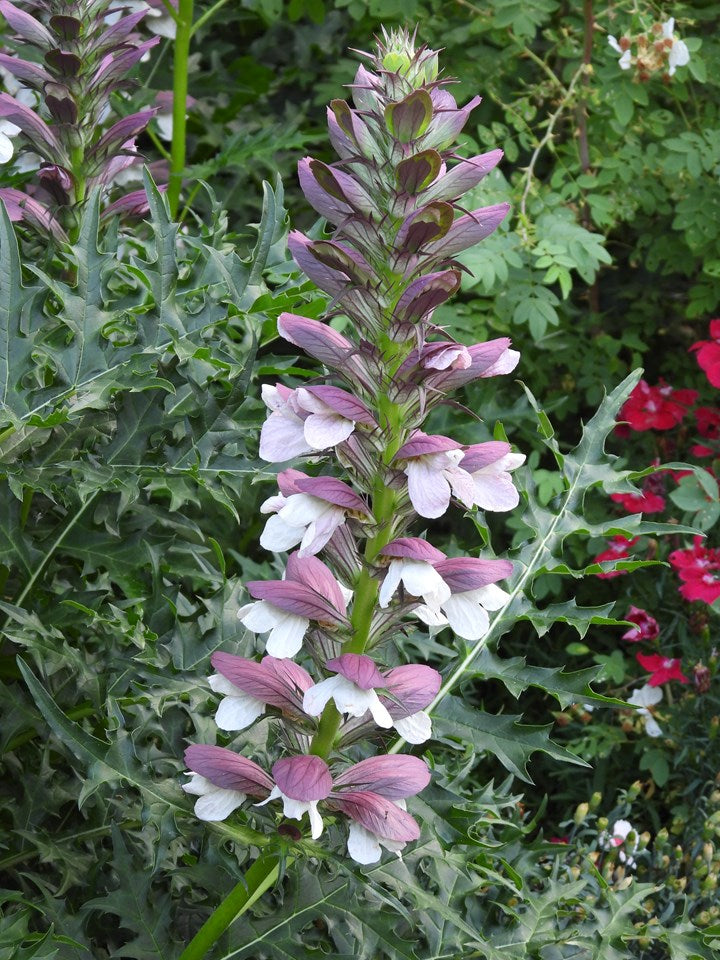This captivating photograph, taken in an outdoor garden, showcases a lush and verdant tropical landscape teeming with diverse vegetation. Dominating the image is a striking plant with a prominent green stalk positioned in the foreground, climbing towards the center-right. This stalk is adorned with alternating purple and white petals, which blossom from the bottom up, creating a mesmerizing cascade of colors. At the base, the flowers are open, revealing deep purple and reddish-purple hues, which gradually transition to tight buds at the top, indicating the plant's blooming progression. The central feature of this plant is a small, tennis ball-sized green bulb, crowned with delicate, fur-like white and purple pollen structures.

Surrounding this central plant, the vibrant greenery envelops the scene, contributing to the image's lush character. To the right, a cluster of pink flowers, resembling forget-me-nots, adds a splash of color, while the top right corner hosts a minute gathering of white flowers with subtle brownish-yellow tinges. The top left is notable for a thick-stalked plant with long, feather-like purple leaves. Throughout the background and foreground, an array of green plants—some with fern-like, spiked leaves resembling children's drawings of Christmas trees—enhances the rich, tropical atmosphere of this serene garden photograph.